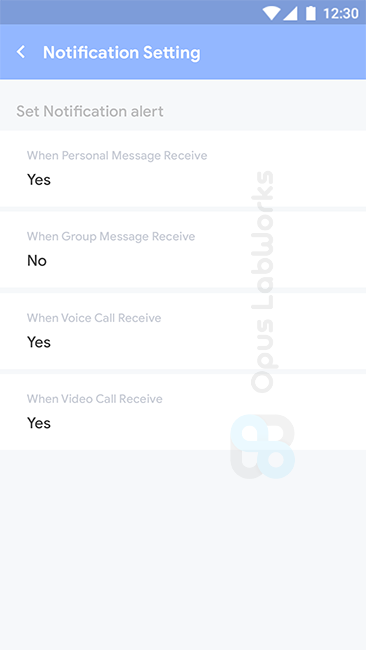The image captures a smartphone screen displaying the Notification Settings page, specifically the section where notification alerts can be customized. At the very top of the screen, there is a thin, horizontal blue rectangle that shows white icons for Wi-Fi, battery status, and the current time, which is 12:30. Below this, a slightly thicker light blue rectangle contains the text "Notification Settings" in white, accompanied by a left-pointing arrow, indicating that this section allows the user to modify alert settings.

The main content of the page lists different types of notifications and their corresponding settings. Indicated by black text, the configuration options are as follows:
- "When personal message received": Yes
- "When group messages received": No
- "When voice call received": Yes
- "When video call received": Yes

Additionally, along the vertical edge of the screen, there appears to be a text, "OPA's lob works," running upward, though it is not entirely clear what this refers to.

Towards the bottom of the screen, there is a large, slightly grayed-out rectangle, which appears blank and might represent a section that is yet to be configured or is currently inactive.